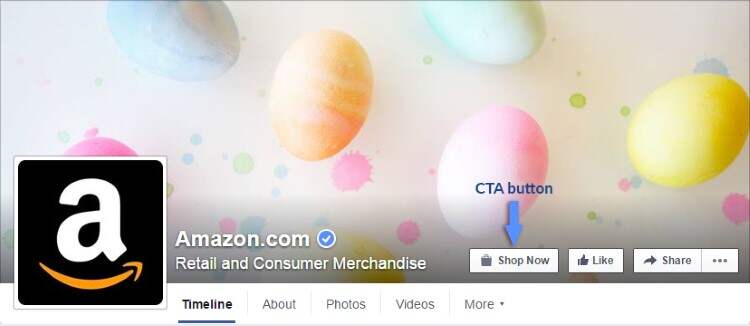This image is a screenshot of what appears to be the top section of an Amazon website. The header occupies a horizontal rectangle, with a white background on the top left gradually darkening towards the right and bottom into a darker gray shade. 

Within this thematic gradient, several Easter eggs are scattered across the area. On the bottom left, partly cropped, is a pink Easter egg. Just above it, slightly to the right, is a blue Easter egg. Central to the image, there's an orange Easter egg adorned with white stripes. Toward the top of the page on the right side, a light green egg is visible, beneath which rests a pink egg that transitions to a lighter hue towards its bottom. Farther right is a yellow Easter egg, which starts as a light yellow on the left and deepens into a mustard color along its bottom and right edges. Additionally, the background features splashes of various paint colors including blue, green, pink, and yellow, which create a festive, colorful backdrop.

In the bottom left corner, occupying about 45% of the width, is a white box with a black background. Inside it, a lowercase white 'a' is accompanied by a yellow right-facing smiley arrow underneath, forming the Amazon logo. To the right of the logo, "Amazon.com" is written in white. Adjacent to this, a blue circle with a white checkmark signifies verification. Beneath this circle, the text "Retail and Consumer Merchandise" is also written in white. 

Further to the right, a "Shop Now" button appears prominently. Positioned above it is the text "CTA button" in blue, along with a bold downward-facing arrow pointing towards the "Shop Now" button. Next to this button are sequentially placed icons and text: a Like button, a Share button, and a Settings button.

Below this header, on the left side, "Timeline" is displayed in bold black letters underlined in dark blue. Following this to the right are "About," "Photos," "Videos," and "More," all in gray letters. The "More" section includes a downward-facing gray arrow, indicating a dropdown menu.